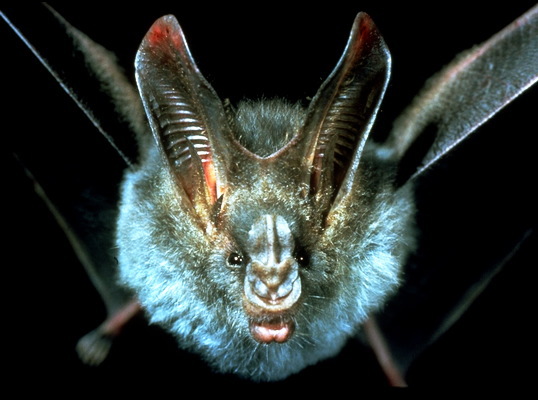This close-up photograph captures a bat in flight, set against a pure black background, providing a striking contrast that highlights the bat's intricate features. The bat, predominantly bluish-white with brown ears and patches along the edges of its wings, dominates the frame. Its face, centered in the foreground with a slightly open mouth revealing small sharp teeth, draws immediate attention. The bat’s large, long ears, which are reddish at the top with horizontal lines running up their brown-hued interiors, stand distinctly upright. The small, black, and bulging eyes add to its expressive appearance. Its face and ears form a sort of circular prominence, with the wings projecting upwards behind. The wings are notable for their black undersides and hints of brown fur on the top side. Blurry, small feet can be seen peeking out below, emphasizing the motion blur of its body. The bat's fur is a mixture of white and brown, with more white tufts concentrated around the face and underside. This image, devoid of any text or background distractions, appears professionally taken, possibly for a nature magazine or an online article, capturing the bat's moment in flight with impressive detail.